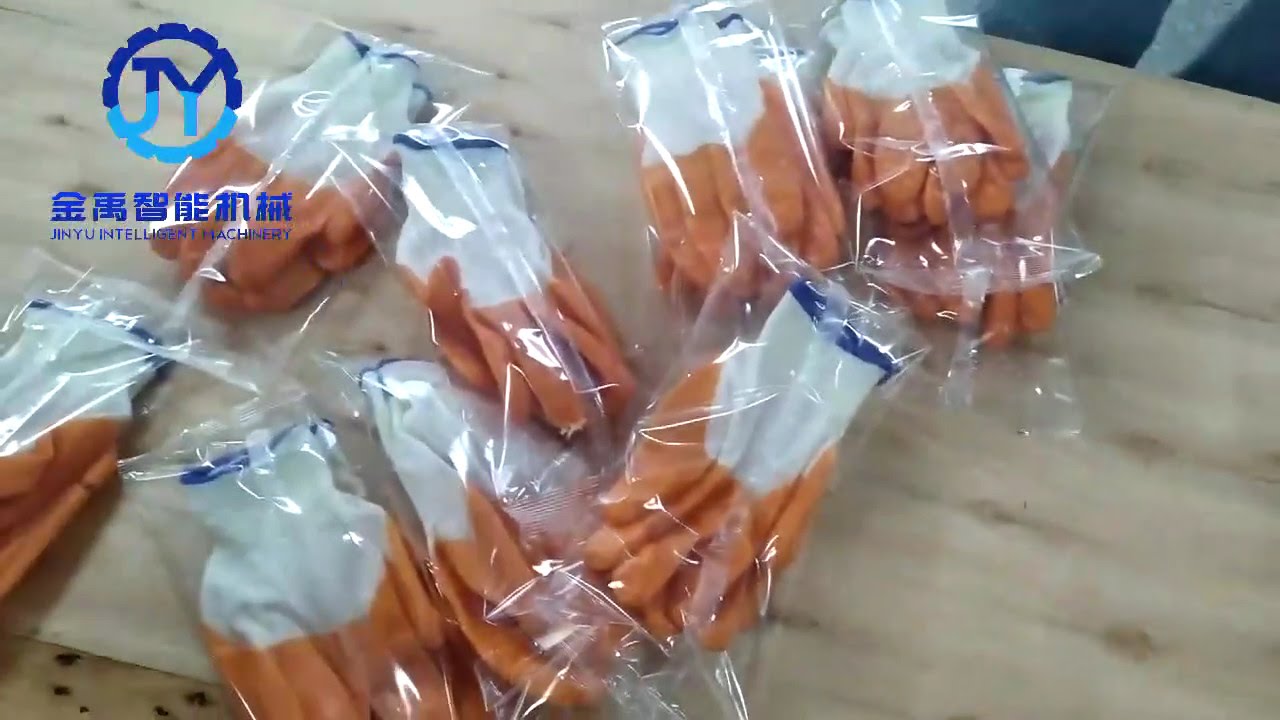This horizontal rectangular image showcases several professionally sealed plastic bags, each containing two pairs of rubber gloves. The gloves feature orange fingers and white palms, with a blue strip near the wrist opening. These bags are neatly arranged on a light tan wooden table, displaying visible wood grain and knots. Notably, there are approximately ten bags on the table.

In the top left corner of the image, a logo with a cog wheel design is visible, displaying the letters "JY" with a gradient from dark blue at the top to light blue at the bottom. Below this logo, Asian characters, likely Chinese or Korean, are present, followed by the English text "Geniu Intelligent Machinery," all written in blue. The background includes a lightly blurred section of beige and brown, hinting at a carpet visible in the top right corner of the image.